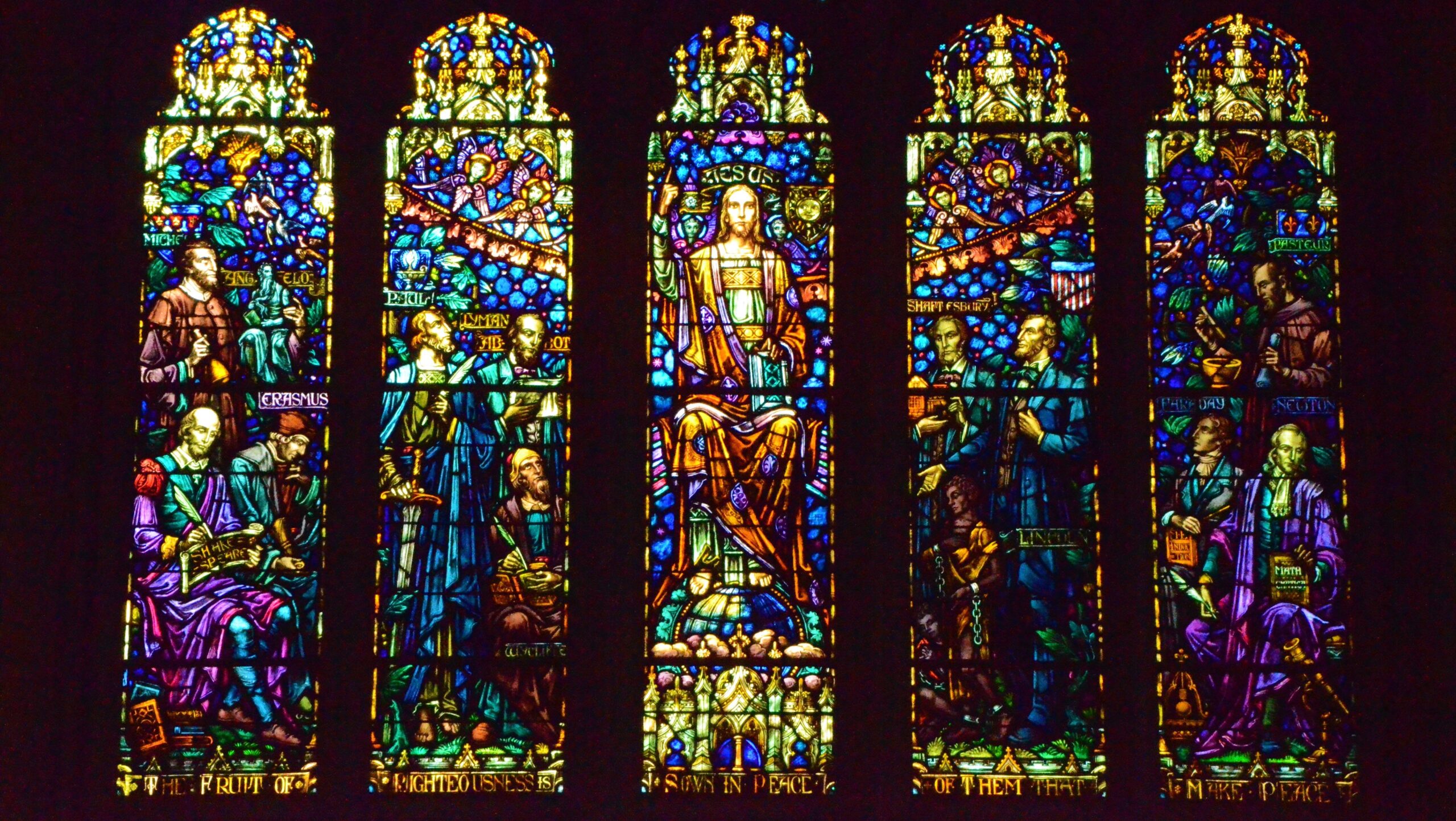This is a photograph of five vertically tall stained glass panels, each with a rectangular base curving into an arched top. These panels are distinctly separated by bold black lines, defining both the windows and the columns between them. Each of the five windows is adorned with vibrant, vivid colors including gold, red, green, purple, yellow, and shades of brown, contributing to a harmonious color scheme across all panels. The stained glass artwork features numerous figures, with some identified by names such as Jesus, Erasmus, Paul, and Abraham Lincoln. The central figure, possibly Jesus depicted with long hair and a robe, is elaborately detailed with blue and purple accents, suggesting a significant and possibly religious context. Surrounding figures on adjacent panels appear to observe the central character, with one on the far left depicted as a scribe, documenting events. The composition suggests a narrative, reinforced by a line of gold text at the bottom of the windows that reads, "The fruit of righteousness sown in peace of them that make peace." The overall artwork exudes a sense of storytelling through its vivid, ornate, and meticulously arranged stained glass imagery.